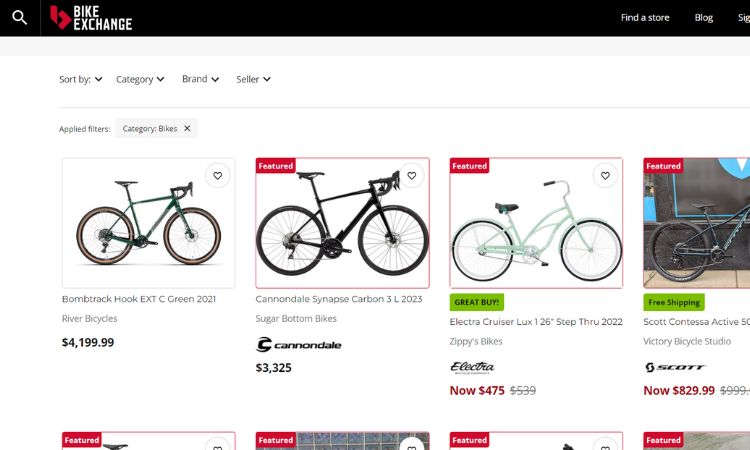Screenshot of the Bike Exchange webpage featuring a sleek black navigation bar across the top, complete with the company's logo and a search option. Below the navigation bar, the screen showcases a selection of available bicycles. Prominently displayed is the Bomb Track Hook EXTC Green 2021 from River Bicycles, priced at $4,199.99. Another notable bike is the Cannondale Synapse Carbon 3L 2023, offered by Sugarbottom Bikes by Cannondale for $3,325. Additionally, the Electra Cruiser Lux 1 26-inch Step Through 2022 from Zippies Bikes by Electra is featured as an attractive option at $475.